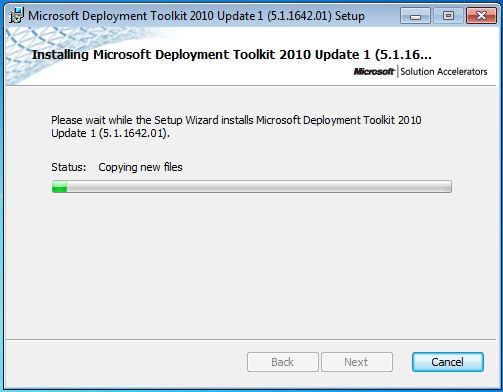The image is a screenshot of a computer screen displaying a typical Windows installation window for the Microsoft Deployment Toolkit 2010 Update 1. At the top of the window, there are standard control buttons: minimize, maximize, and close (red X). The window header reads "Microsoft Deployment Toolkit 2010 Update 1." The main section of the window, which has a gray background, prominently displays the text: "Please wait while the setup wizard installs Microsoft Deployment Toolkit 2010 Update 1." Below this, it shows the status message "copying new files" alongside a partially filled progress bar that indicates the installation is about 5-10% complete with a small section in green. At the bottom of the window, there are three buttons: Back, Next, and Cancel. The Back and Next buttons are grayed out and unclickable, while the Cancel button is highlighted in blue, indicating it is the only actionable option at this stage. Additional labeling includes "Microsoft Solution Accelerators."